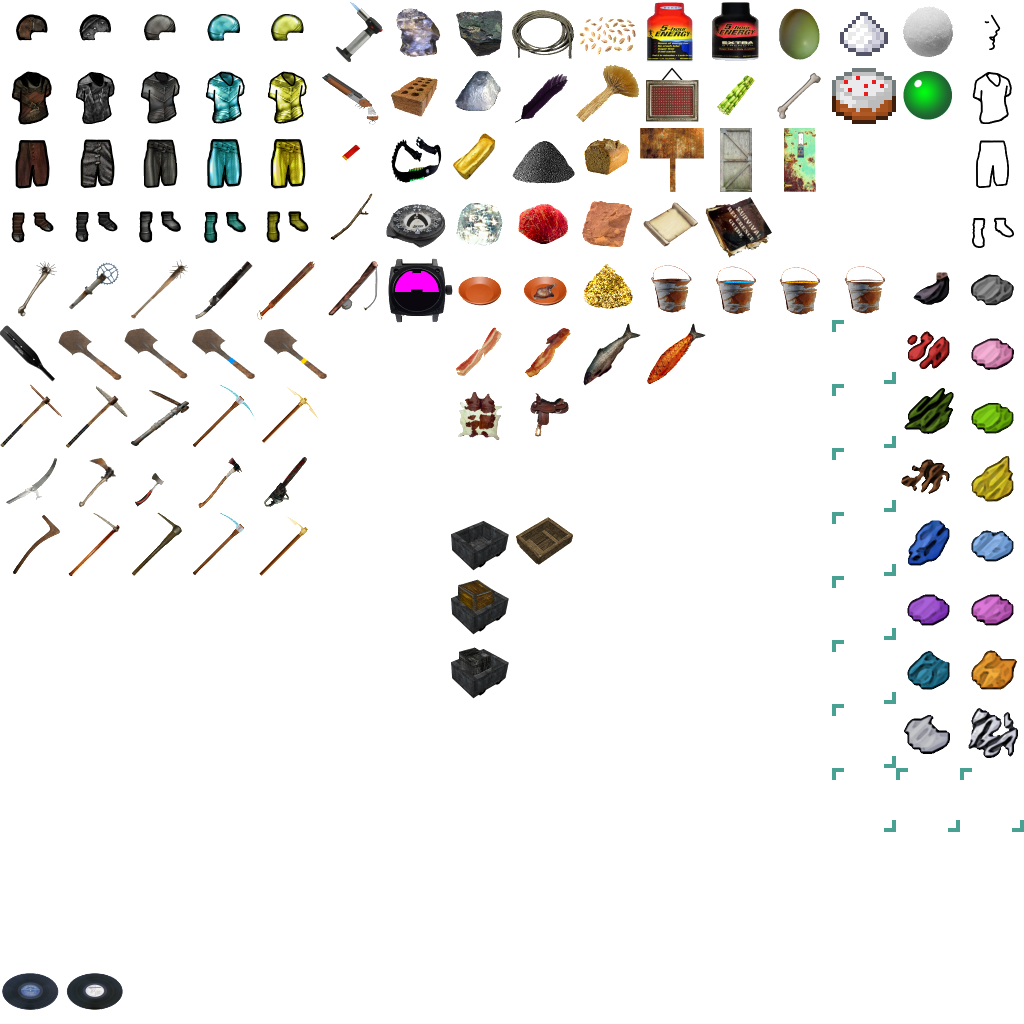The image depicts what appears to be an inventory screen from a video game, characterized by 12 rows of icons and two smaller end rows featuring L-shaped dashes and X-shapes. The first row showcases various helmets and miscellaneous items, including what might be 5-hour energy bottles. The second row includes shirt icons, some symbols such as bricks and hammers, and perhaps a dog bone, along with other indistinguishable objects like pictures, cakes, and balls. The third row has an assortment of pants in brown, gray, blue, and yellow hues.

The fourth row houses different colored shoes on the left and ambiguous square icons on the right, in shades of red and silver. The fifth row consists of tools on the left, containers or buckets on the right, and a pink item with a disc inside in the middle, along with a bagel-like brown object without a hole. The sixth row features shovels and tools on the left, fish in the middle, and jagged, colorful items in red and purple hues on the right.

Axes dominate the left side of the seventh and subsequent rows, with various items like brown and gray boxes in the middle and colorful, rock-like objects on the right, ranging from blue and light blue to pink, purple, and white. The inventory screen includes a mix of realistic items like bricks and lighters and more cartoonish, animated items resembling those in games like Minecraft. The image serves as a comprehensive table of contents for the game's inventory, covering clothing, weapons, tools, food, and minerals. At the very bottom, separated from the main rows, are two record discs seemingly meant for playback.